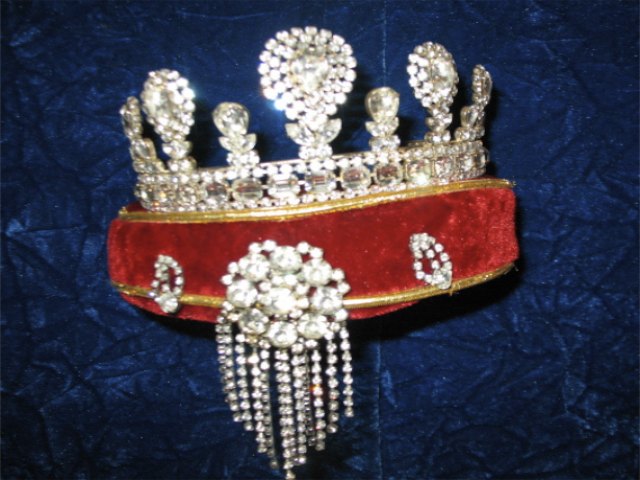The photograph captures an opulent crown seemingly floating on its display, set against a luxuriously wrinkled, soft velvety blue background. The crown itself is a round velvet hat adorned with intricate gold embroidery along both the top and bottom edges. A notable feature at the front includes two circles of diamonds dangling elegantly, complemented in the center by a larger diamond shape from which multiple diamond chains cascade. The crown’s top is encircled by a band of gold and diamonds, punctuated at random intervals by delicate diamond flowers. All of these elements together create a stunning and regal piece, exuding a royal aura with its rich colors and lavish detailing.